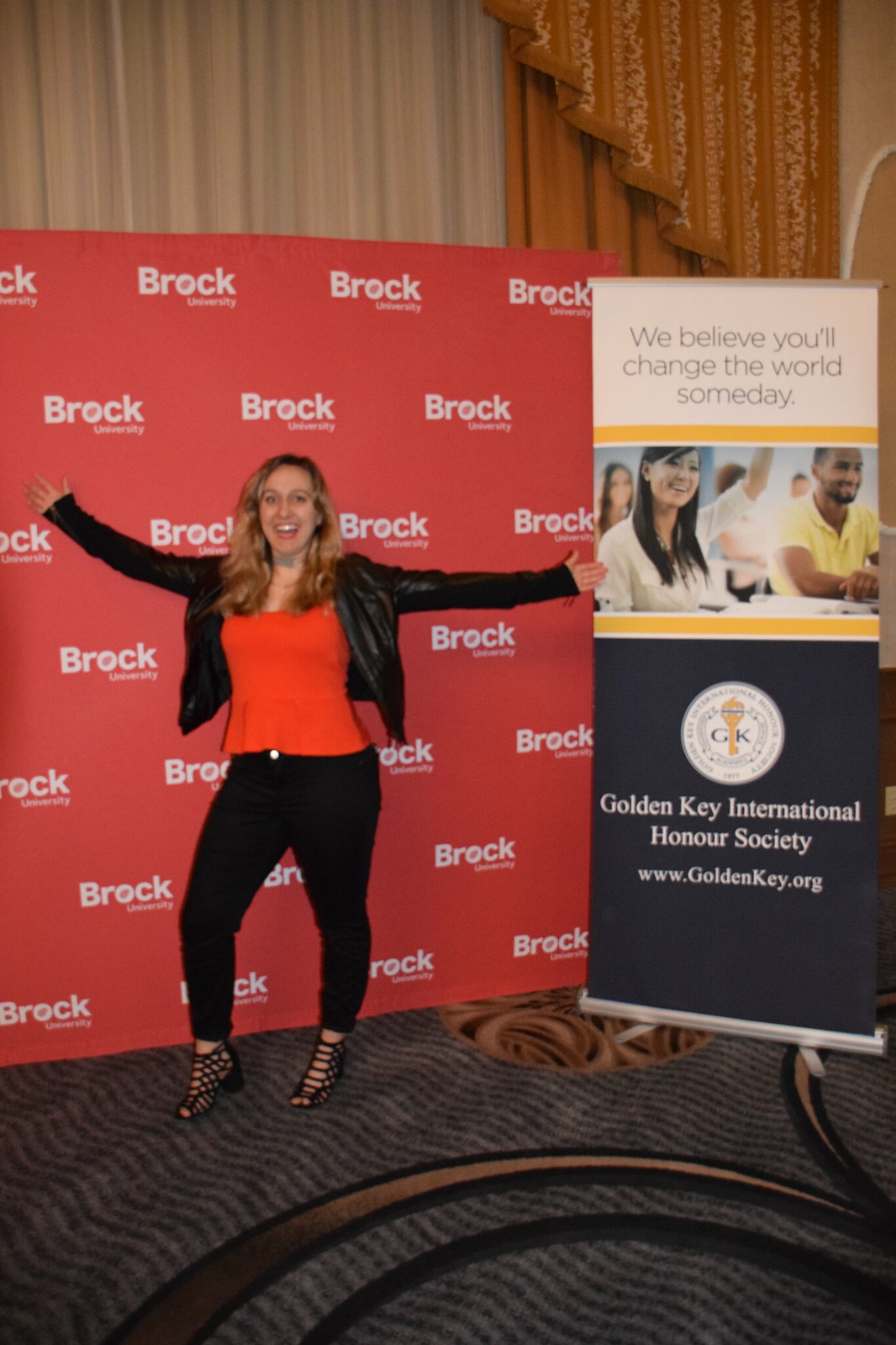In a photograph taken at a convention, a woman with shoulder-length, light brown hair is smiling and posing for the camera. She is dressed in a black leather jacket, a red shirt, black pants, and strappy high heel shoes. The woman stands on a gray, wavy carpet, arms outstretched on either side, in what appears to be a hotel conference room or banquet hall, characterized by grand curtains. Behind her, there is a red backdrop with the repeated white logo of Brock University. To her right stands a tall banner reading, "We Believe You'll Change the World Someday," along with the text, "Golden Key International Honor Society www.goldenkey.org" and a logo featuring "GK" with a key. The overall atmosphere is professional, accentuated by the carpeted floor and formal backdrop emphasizing the educational and motivational event.